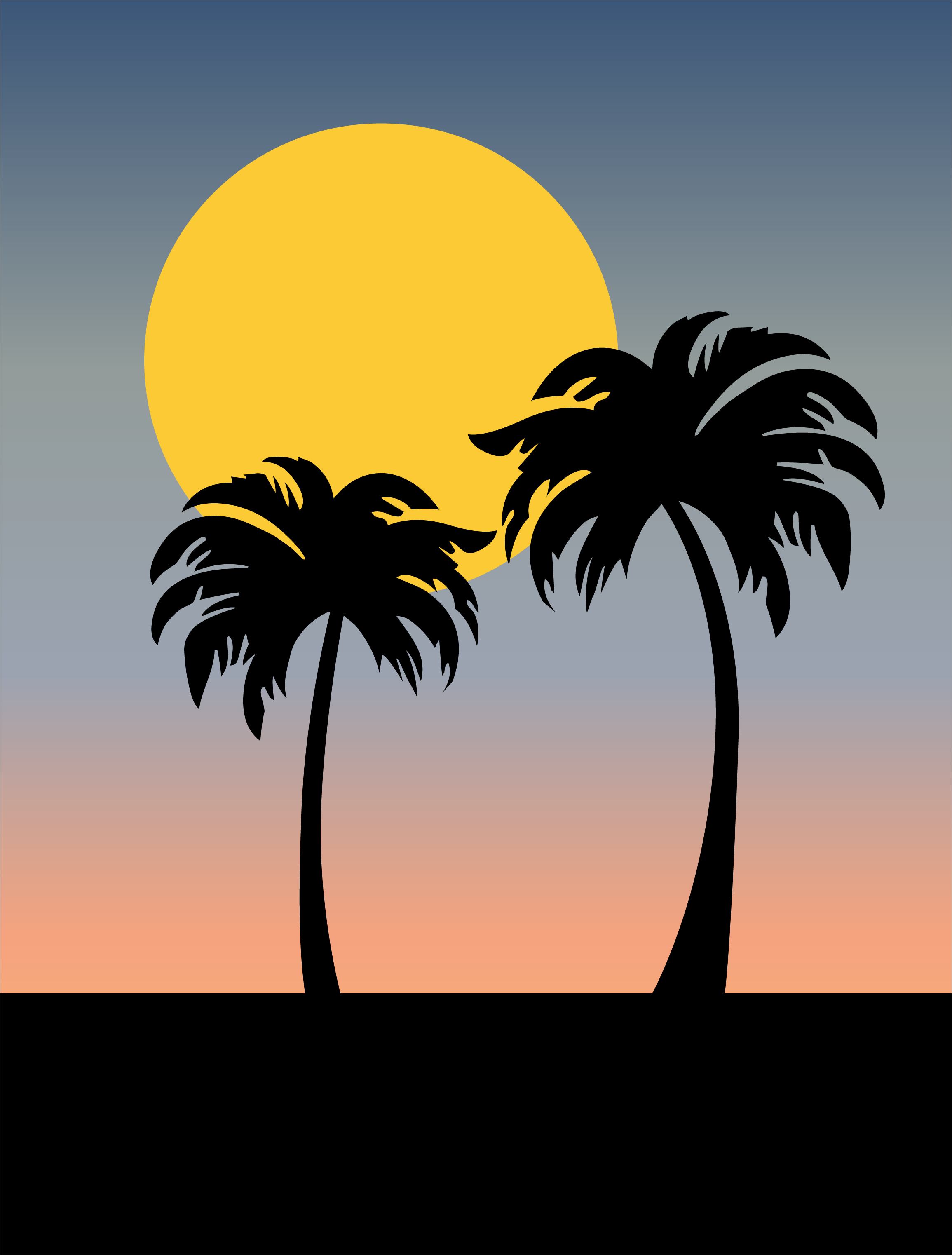This illustration depicts the striking silhouettes of two palm trees rising from a flat black rectangle at the base. The palm trees are stark black, with the tree on the right marginally taller than the one on the left. Their detailed leaves partially overlap a prominent, flat yellow circle representing the sun, which sits just above them. The background is a mesmerizing gradient that transitions from a deep peach color near the horizon to bluish-gray at the top, giving the appearance of a sunset sky. The entire scene is rendered in simple, yet striking pastel hues, creating a serene and minimalist landscape.